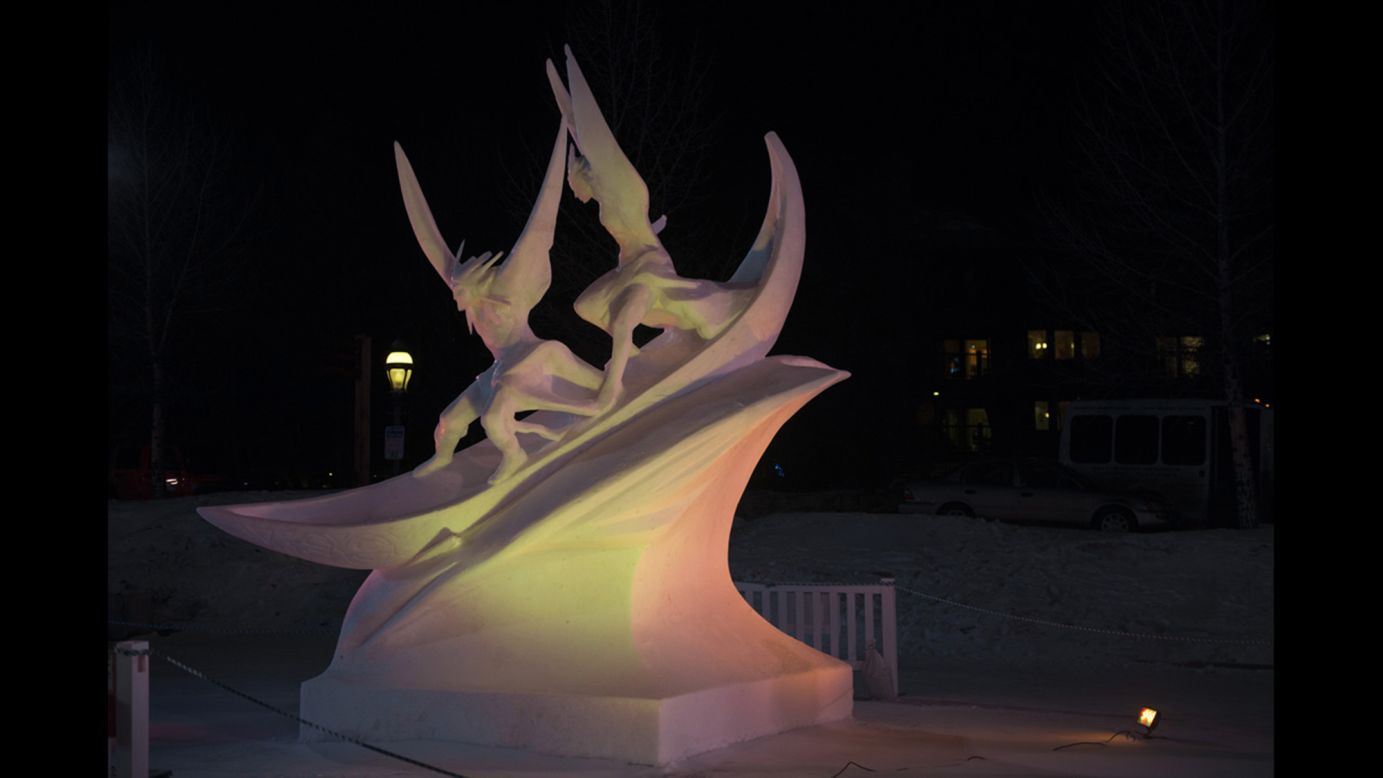This nighttime color photograph showcases a stunning snow sculpture, meticulously framed and protected by chains and posts at its base. Illuminated with vibrant hues of green and red, the sculpture stands on a square pedestal, drawing attention to its intricate design. Emerging from the bottom left of the pedestal is a dynamic, curving form that evokes the movement of a wave. Riding atop this wave is a detailed representation of a canoe with two figures, their arms raised in exuberance as they appear to glide effortlessly. The dark, expansive sky in the background, dotted with distant lights, contrasts sharply with the vivid illumination of the sculpture, accentuating its details. The photograph’s landscape orientation further emphasizes the breadth of the scene, capturing a moment of frozen artistry in vivid detail.